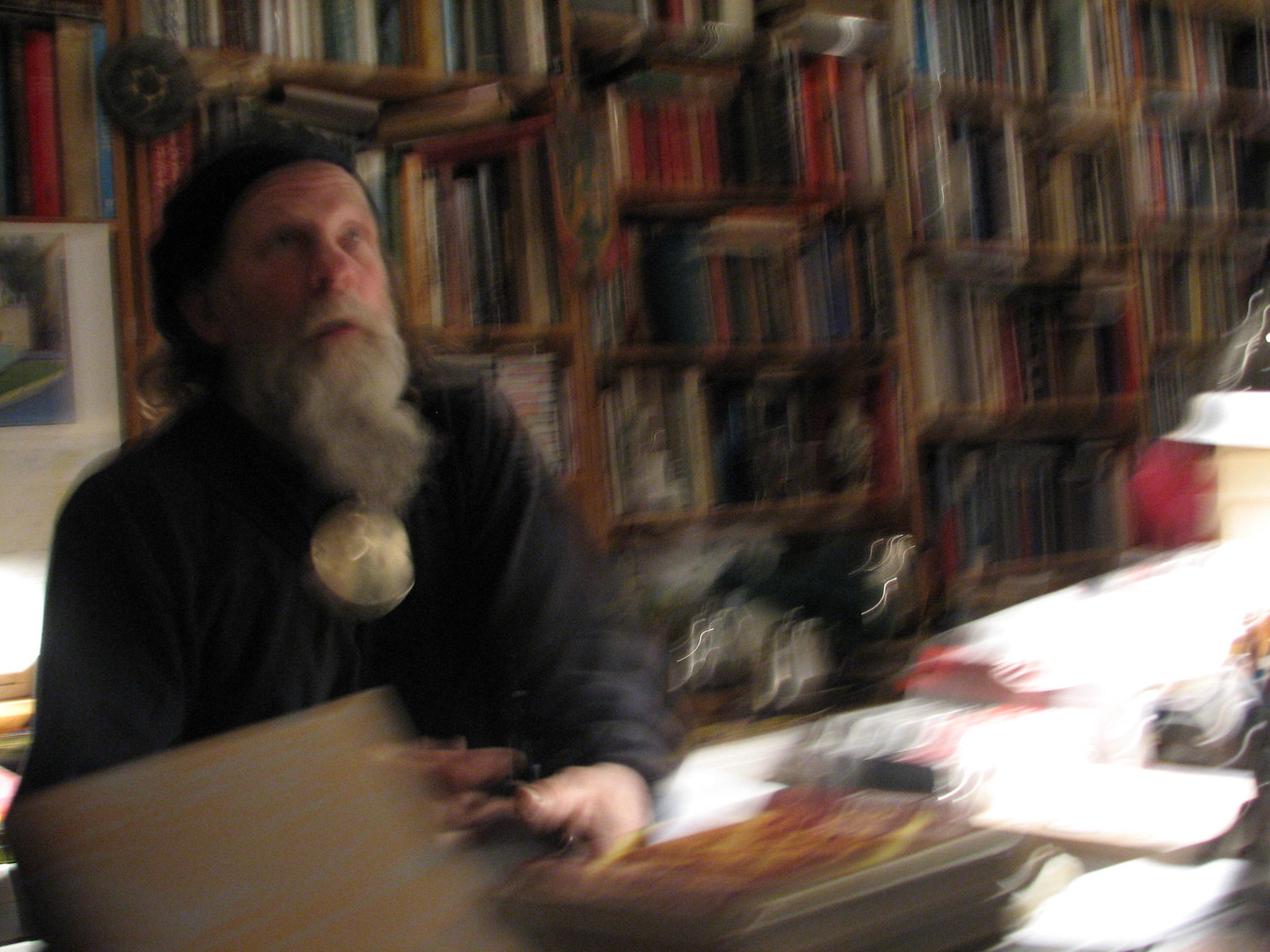In this slightly blurry photograph, an older Caucasian man with a long gray beard and possibly long hair tied back is the focal point. He’s wearing a black long-sleeve shirt or tunic, with a bronze or gold medallion around his neck, and a black hat or headscarf. The man is seated at a brown desk cluttered with books and materials, and he's looking upward towards something off-frame. Behind him, the background is filled with large, solid bookcases packed with hundreds of books of various colors, dominated by reds, blues, and greens. The setting appears to be a study room or library, dimly lit, perhaps by the soft glow of a desk lamp. There’s also a portrait and some medallions decorating the space, adding to the cozy, intellectual ambiance of the scene.